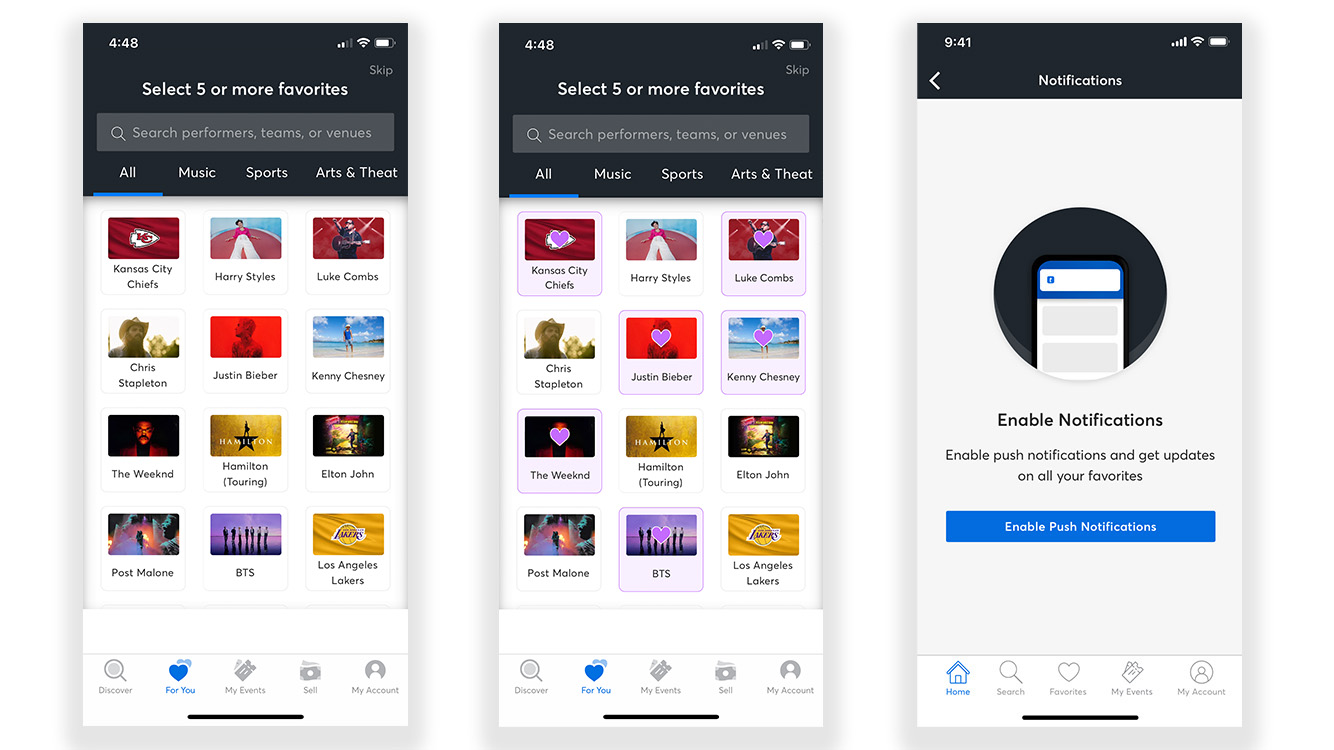Here is a detailed and cleaned-up caption for the series of screenshots described:

---

The series of images consists of three screenshots captured from an iPhone within a music application. 

**First Screenshot:**
The interface displays several UI elements:
- **Status Bar:** Located at the top, with a black background. The time shows as 4:48 in the upper left corner. The far-right corner shows the signal strength with two out of four bars in white, a fully white Wi-Fi icon, and a partially white battery icon.
- **Skip Option:** In light gray text beneath the status bar.
- **Instruction Text:** Centered in white text, "Select five or more favorites."
- **Search Bar:** A dark gray bar with a magnifying glass icon and placeholder text, "Search performers, teams, or venues."
- **Categories:** Four options in white text - "All," "Music," "Sports," and "Arts & Theater." Only "All" is selected, indicated by a blue underline.
- **Selection Grid:** Four rows, each with three options:
  - 1st Row: Kansas City Chiefs, Harry Styles, Luke Combs
  - 2nd Row: Chris Stapleton, Justin Bieber, Kenny Chesney
  - 3rd Row: The Weeknd, Hamilton (Touring), Elton John
  - 4th Row: Post Malone, BTS, Los Angeles Lakers
- **Bottom Navigation Bar:** Five icons - a magnifying glass ("Discover"), a heart ("For You," highlighted in blue), a ticket ("My Events"), what appears to be a file ("Self," or similar), and a silhouette ("My Account"). Each icon has associated text labels.

**Second Screenshot:**
Similar layout to the first with some selections made:
- **Selected Items:** Kansas City Chiefs, Luke Combs, Justin Bieber, Kenny Chesney, The Weeknd, and BTS. These selected items are highlighted with a light pink outlined box.

**Third Screenshot:**
The interface changes to a notification settings screen:
- **Status Bar:** Time now shows 9:41 in the upper left corner. The far-right corner shows full signal bars, the Wi-Fi icon, and battery icon.
- **Toolbar:** A back arrow on the upper left and centered text "Notifications."
- **Main Body:** White background with a central black circle featuring an iPhone icon. Below it is the text, "Enable Notifications. Enable Push Notifications to get updates on all your favorites." 
- **Enable Button:** Blue box with white text, "Enable Push Notifications."
- **Bottom Navigation Bar:** Icons similar to the previous ones, with "Home" (house icon) now highlighted in blue, alongside Search, Favorites, My Events, and My Account.
- **Common Feature:** A black line appears at the bottom center of each screenshot.

---